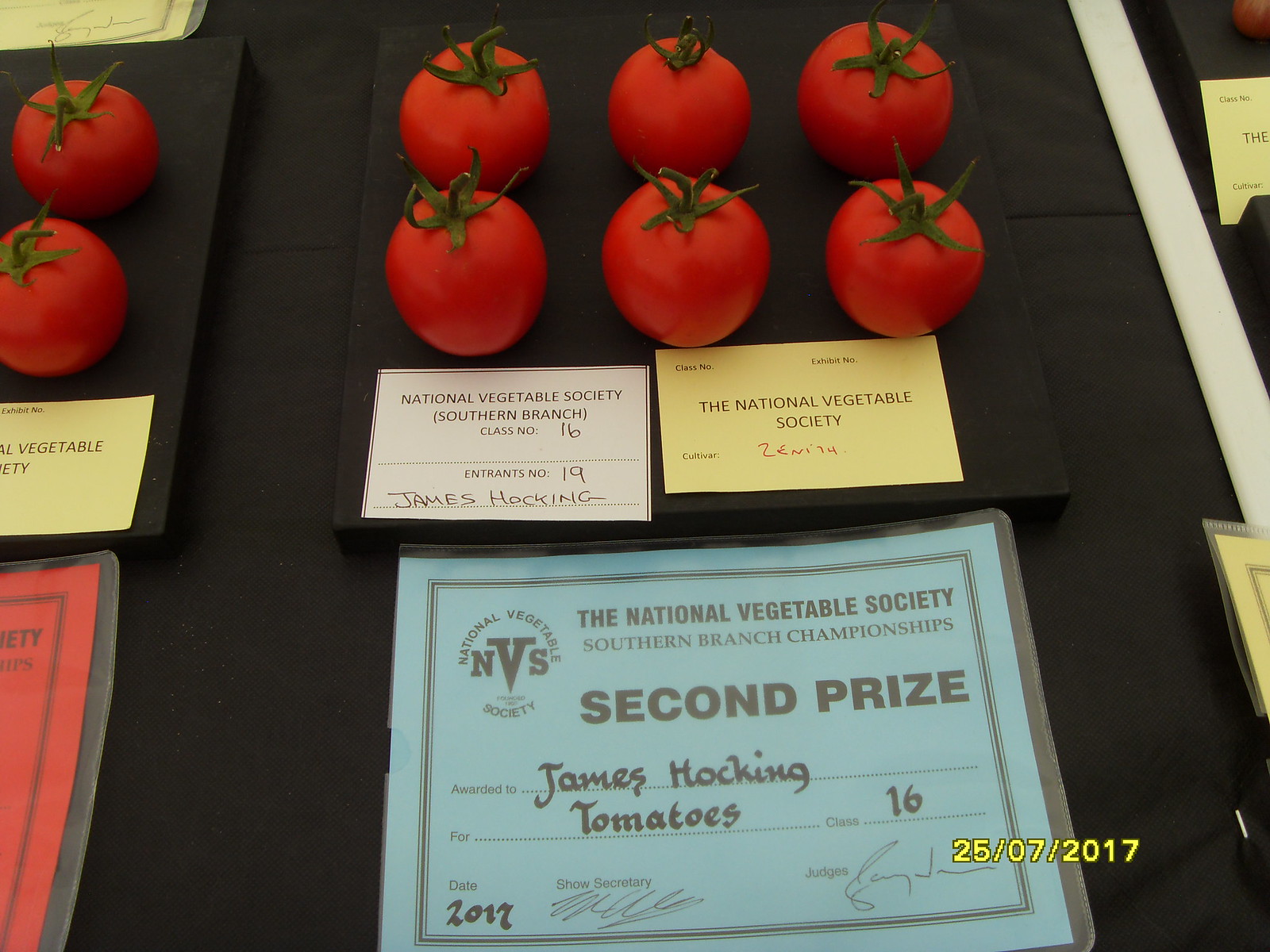The image captures a vibrant display of competition-grade tomatoes, set against a black fabric surface. At the center top of the image, a black square-shaped platform showcases six vibrant red tomatoes, each with healthy green stems and leaves, meticulously arranged in two rows of three. A partially visible, identical platform appears on the left. Prominent signs are placed prominently below the tomatoes; a white rectangular sign features the text "National Vegetable Society, Southern Branch, Class No. 16, Entrance No. 19, James Hawking." Adjacent to it, a yellow rectangular card simply states "The National Vegetable Society." Below these signs, a laminated blue piece of paper reads, "The National Vegetable Society, Southern Branch Championships, Second Prize, James Hawking for Tomatoes, Class 16, 25/07/2017." The overall presentation highlights James Hawking's achievement in this prestigious Southern Branch vegetable competition.